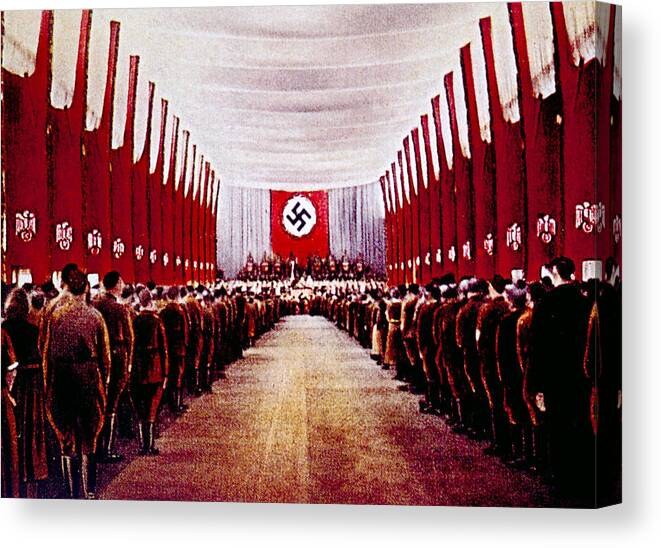This detailed vintage image, either a photograph or painting, depicts a Nazi rally during World War II. The focal point is a large red flag displaying a black swastika within a white circle, hanging prominently in the background. The scene is set in what appears to be a large auditorium or meeting facility adorned with white drapery on the ceiling. 

There is a clear aisle running down the middle of the room, bordered by rows of soldiers in brown uniforms and high black boots, standing at attention. The soldiers, aligned on both sides of the path, are facing forward towards the stage and listening intently to a speech, though the speaker is not visible due to the distance. Flanking the walkway are numerous red banners, some appearing to depict the German coat of arms, an eagle symbol.

The overall color palette includes reds, browns, and blacks, giving the image an intense and somewhat grainy, recolored feel. The scene captures a moment of strict attention and order during the Nazi regime, with a dense crowd emphasizing the scale and solemnity of the gathering.